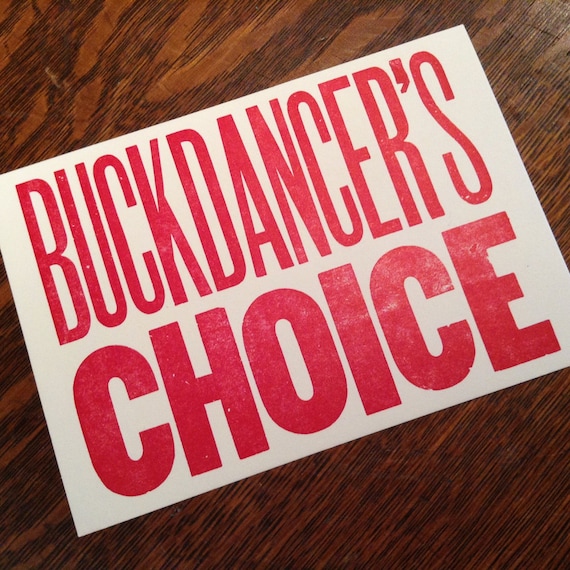This photograph features a rectangular sign with prominent red text on a white background, positioned at a slight angle on a dark brown wooden table. The table's wood grain is distinctly visible, marked by some black streaks. The text on the sign reads "BUCK DANCER'S" in a thinner, bold, all-caps font stretched to fit across the width, followed by the word "CHOICE" in a thicker, blockier font, also in bold, all-capital letters. The sign's cleanly cut edges contribute to its neat presentation.